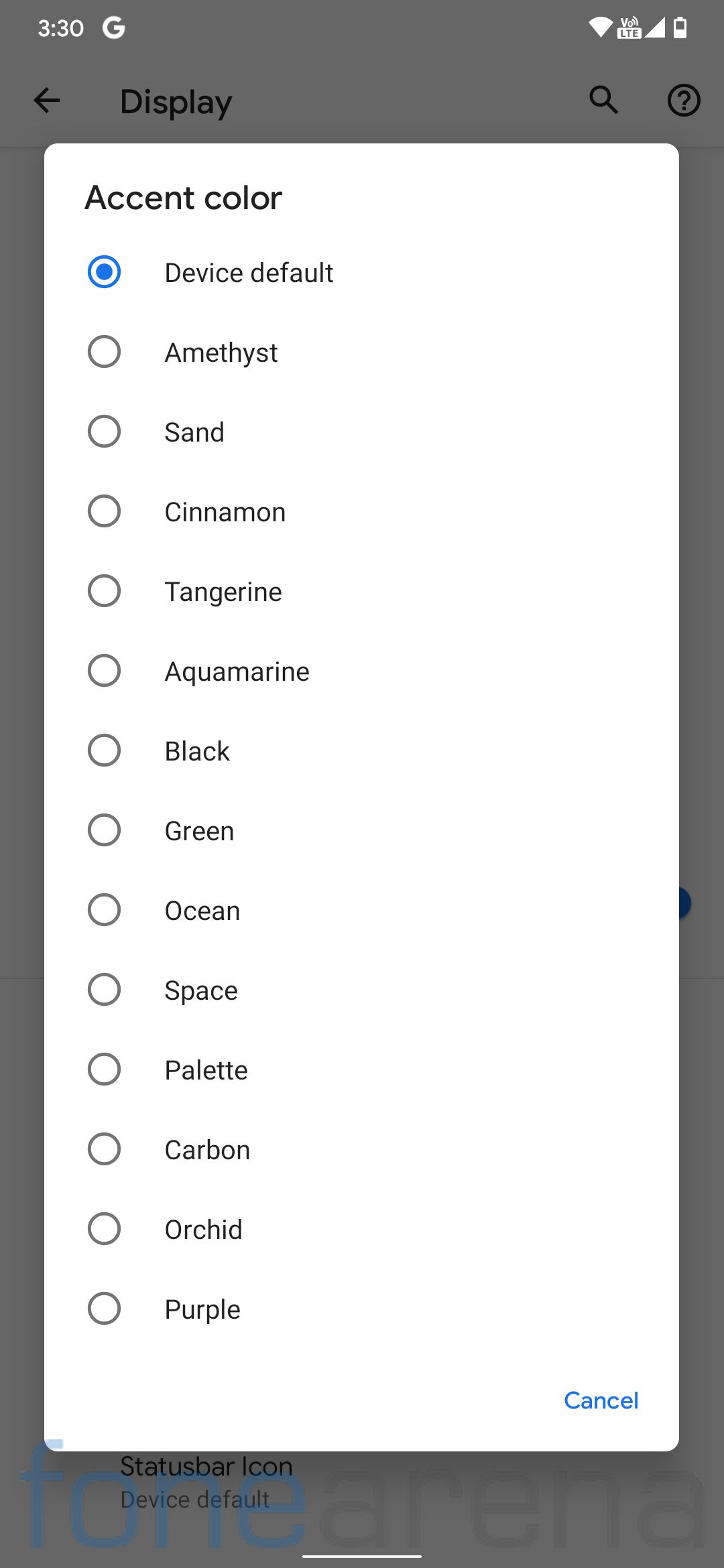This is a detailed and cleaned-up caption for the described screenshot:

---

A screenshot showcasing a settings menu with a gray background at the top, displaying the label "333" or "330 G," an arrow symbol pointing backward, a battery icon, and a black question mark icon next to a black search bar. The section is labeled "Accent Color" with the option "Device Default" checked off. Available color choices include Amethyst, Sand, Cinnamon, Tangerine, Black, Green, Ocean, Space, Pallet, Carbon, Orchid, and Purple. Below the "Accent Color" section, there is a "Suspension Bar Icon" label. Accompanying this label, some words appear in blue text, though they are illegible. The interface features a cancel button, with the left section of the screen in white and the right section in black.